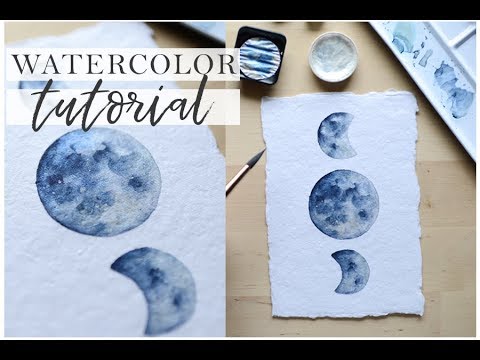This advertisement features a watercolor tutorial prominently displayed in black font against a white background at the top left corner. The image is bordered by horizontal black bars at both the top and bottom. Central to the photo is a light-colored wooden table holding two sheets of white paper, each showcasing different moon phase paintings rendered in various shades of blue and gray.

The left sheet displays a full moon above a crescent moon. Just behind this paper, partially obscured, is a watercolor paintbrush. The right sheet features another series of moon phases: a full moon at the center, flanked by a right-facing crescent moon on top and a left-facing crescent moon on the bottom. Positioned in the top right corner of the table lies a watercolor tray, essential for the tutorial. The composition of the ad not only highlights the artistic elements but also aligns them in a neat, visually appealing arrangement.